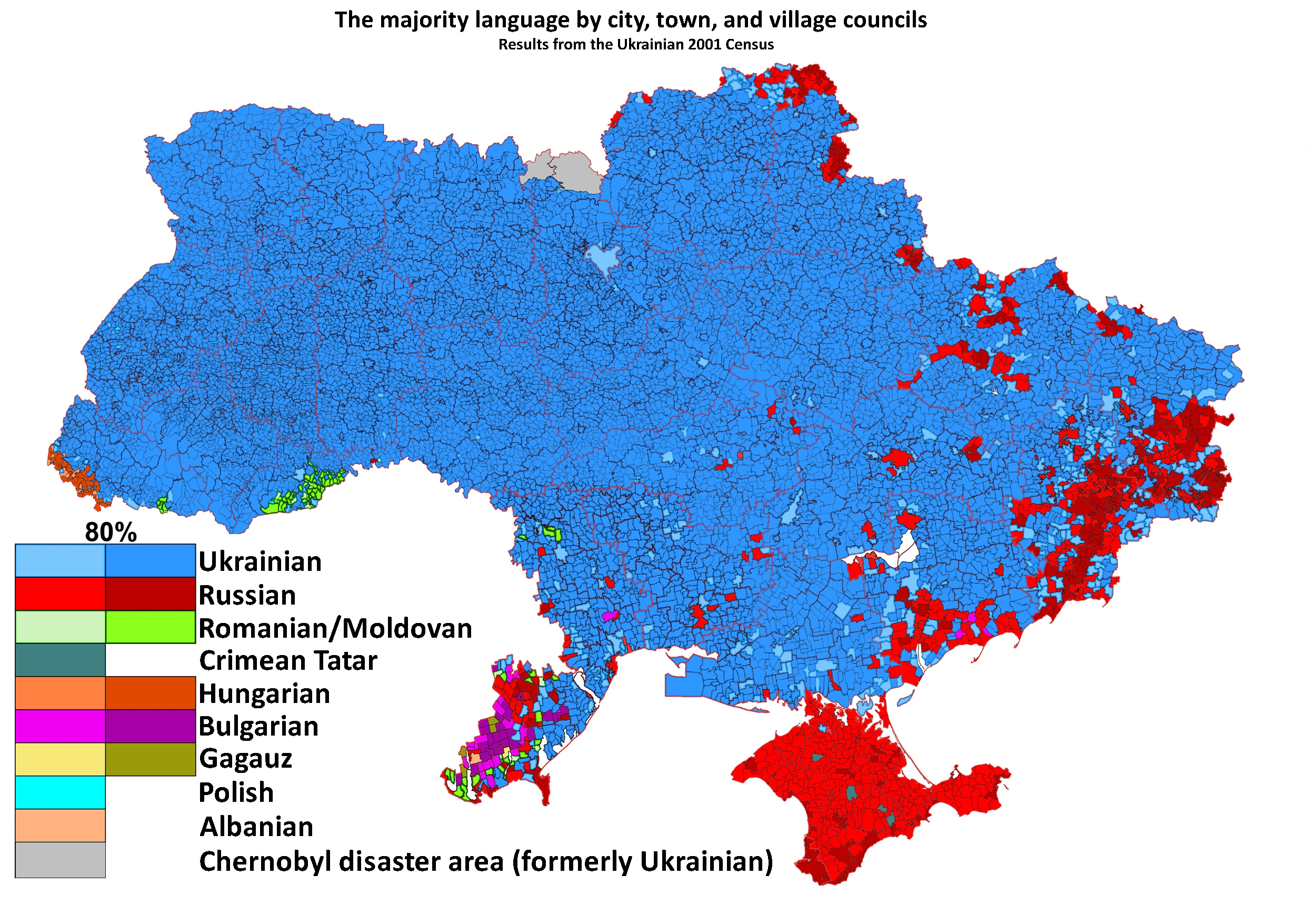This image is a detailed map predominantly covering Ukraine, titled "Majority Language by City, Town, and Village Councils" based on the results from the Ukrainian 2001 Census. The map features various regions color-coded to represent the majority languages spoken in each area. The majority of the map is colored in medium blue, indicating that Ukrainian is the predominant language spoken in about 80% of the depicted regions. 

Along one coast, there are patches of green in two shades—a lighter green and a slightly darker green—which signify areas where Romanian and Moldovan (or Moldovian) are spoken. The next most prominent color on the map is red, indicating regions where Russian is the majority language. There are also other minor languages depicted on the map, but they occupy much smaller areas compared to the dominant blue regions representing Ukrainian speakers. 

This detailed linguistic distribution map provides a comprehensive visual representation of the primary languages spoken across various municipalities in Ukraine as of 2001.